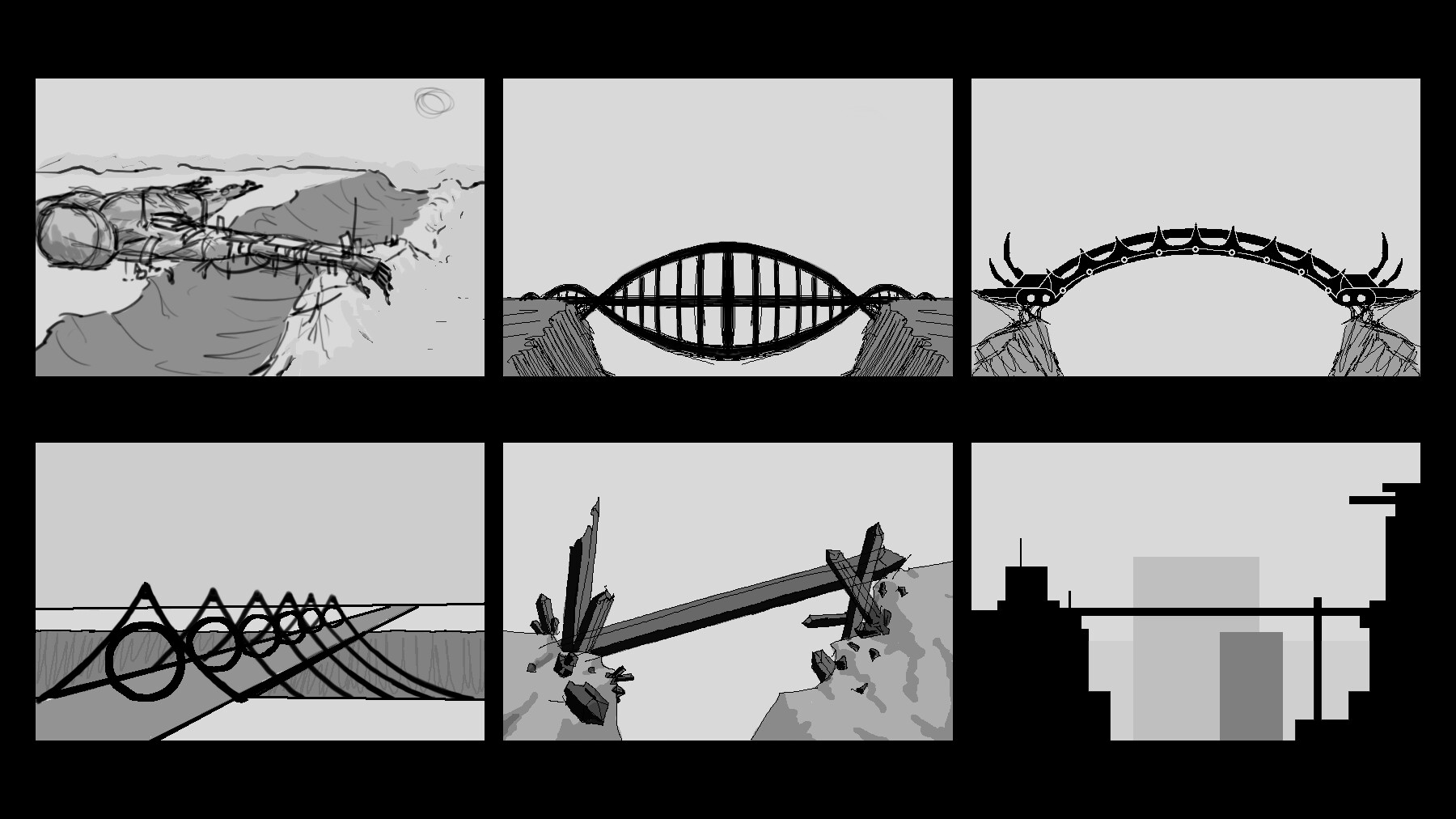The image is a black and white, six-frame collection showcasing various bridge designs traversing chasms and valleys. Each frame is distinct, yet they share a unified aesthetic of stark contrast. 

In the top left frame, a roughly sketched bridge crossing a natural canyon is displayed, with ambiguous materials suggesting a sturdy yet raw structure, possibly a fallen tree. The top center frame features an ornate ironwork bridge with a semicircular design and decorative end caps, spanning a similar canyon and reflecting a fantasy-style construction. The top right frame exhibits an arched bridge with a striking, almost scorpion-like silhouette, elegantly crossing a deep ravine.

Descending to the bottom row, the lower left frame portrays a fanciful bridge constructed of triangular arches and straight walkways, supported by suspension ropes, extending away from the viewer across a canyon. The bottom center frame shows a crudely assembled bridge made from wired-together wooden planks, spanning a chasm with irregular ends. Finally, the bottom right frame presents a simplistic cityscape with basic block shapes, featuring a thin metal bridge that connects two buildings, creating a stark juxtaposition within a minimalistic urban skyline.

Heavy black borders frame the entire collection, emphasizing the visual cohesion of these diverse and imaginative bridge designs.